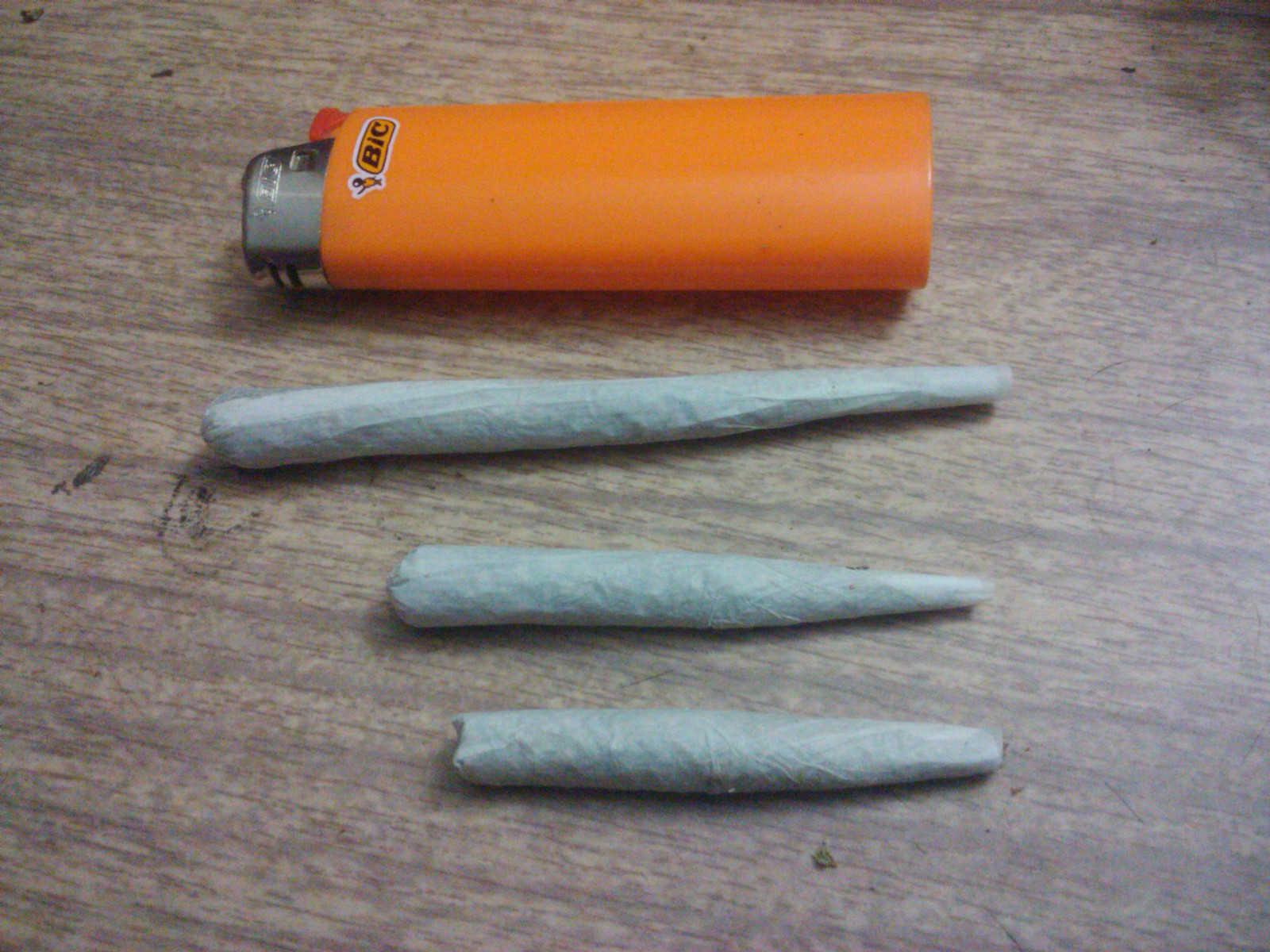This square color photograph showcases an orange disposable Bic lighter positioned in the top quarter of the frame, set against a grainy, light brown wooden background with hints of gray. Below the lighter are three hand-rolled cigarettes arranged in descending order of size. The top cigarette is the longest, the middle one is slightly shorter and slightly fatter, and the bottom one is the shortest and fattest. These cigarettes are wrapped in gray paper, and their exact contents are unknown. The scene includes some black markings to the left of the longest cigarette and small bits of dirt or debris near the bottom one. The lighter features "BIC" written in black on a yellow background with a white outline and a black border, and has a red ignition button.